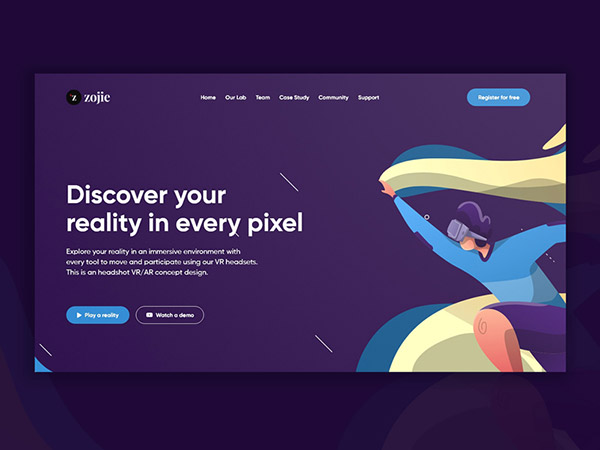"Explore a new realm in every pixel. In the left scene, a person is depicted holding a blanket with a virtual reality headset on, immersed in a digital experience. Similarly, on the right, another individual is engaged in a virtual world, blanket in hand and headset firmly in place. This juxtaposition captures the captivating blend of technology and everyday life, inviting you to 'play' your reality and watch it unfold in the virtual domain."